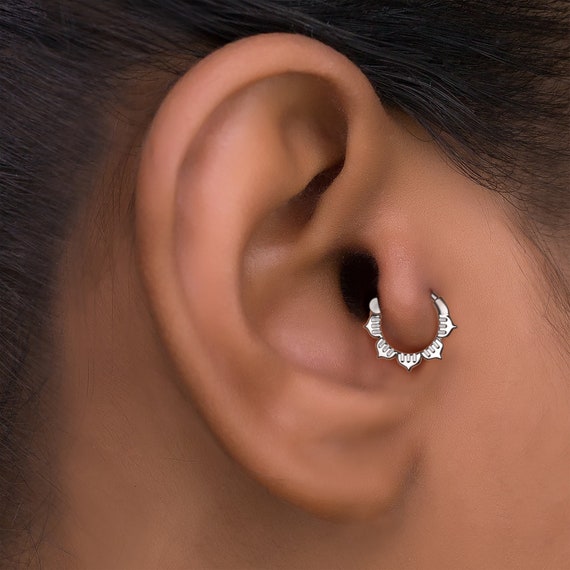This close-up image highlights a beautifully intricate tragus earring adorning a woman's ear with tan or olive-colored skin and dark brown, pulled-back hair. The earring is a dainty, circular piece made of silver or stainless steel, featuring five pointed, curved, delicate adornments that resemble pointed droplets forming the inverted roof of a small cathedral. The tiny, flower-patterned tragus earring is precisely pierced through the small knob of cartilage that projects from the ear canal. The ear and hair are the main focus, with no discernible background, emphasizing the earring's shiny and delicate design. The overall presentation suggests a product showcase, emphasizing the elegance and subtleties of the piercing.